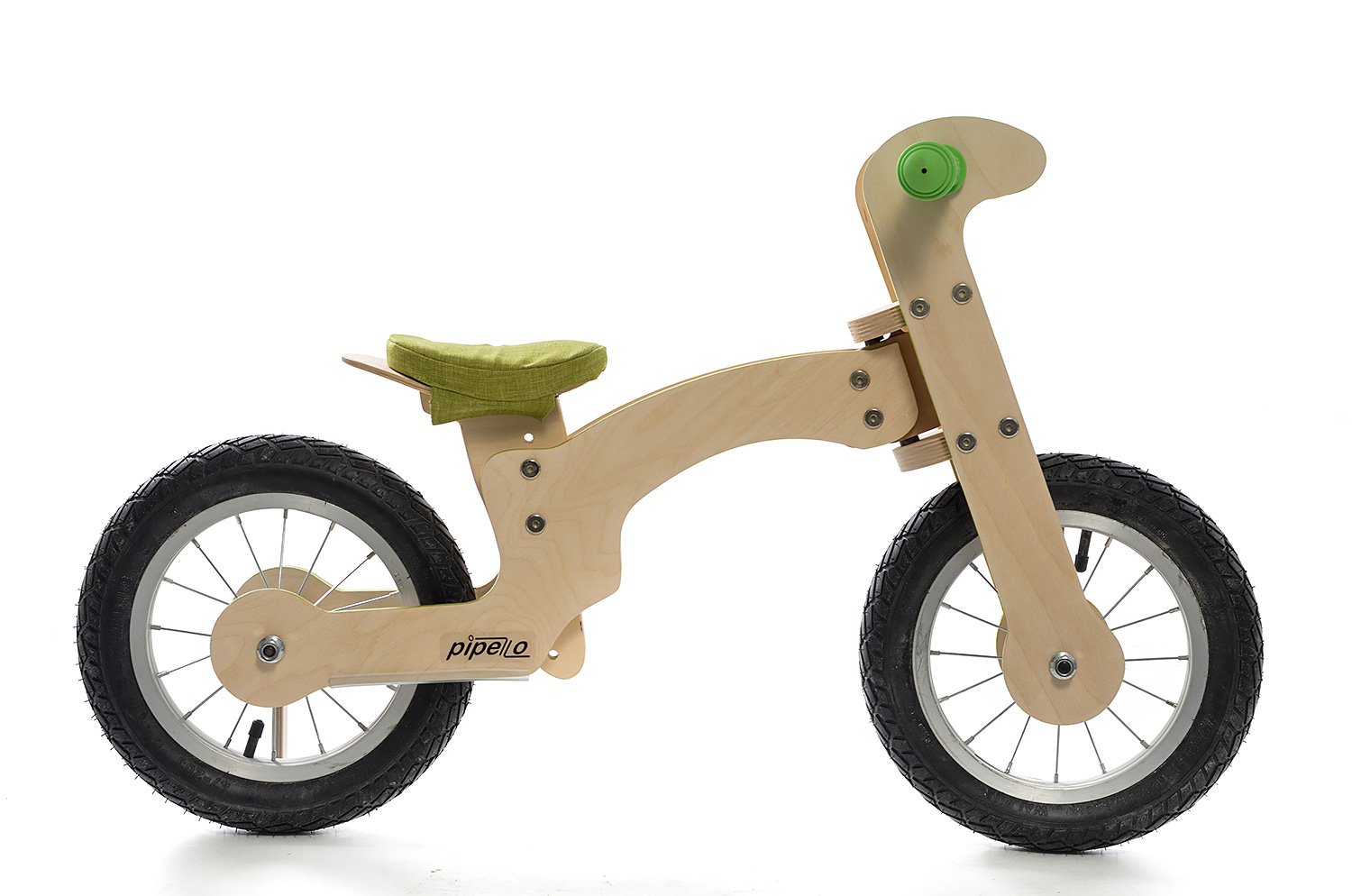This is a detailed side view product image of a small wooden child's kick bike, set against a completely white background and professionally lit to highlight the item's features. The bike, designed for young children up to five or six years old to help them learn balance, has a thin, light wooden frame. It features a soft, removable green cushioned seat and green plastic handlebars for the child to grip. Both the front and back tires are made of thick, black rubber with prominent treads and are mounted on silver wheels with spokes. The front forks and the structure of the handlebars are also wooden. Noticeable screws are visible along the joints of the bike, emphasizing its assembled nature. Additionally, the bottom left of the bike near the rear wheel features the 'Pepello' logo, presumably the brand. This high-quality rendering is likely intended for use in a store's website or a magazine advertisement to promote the product.